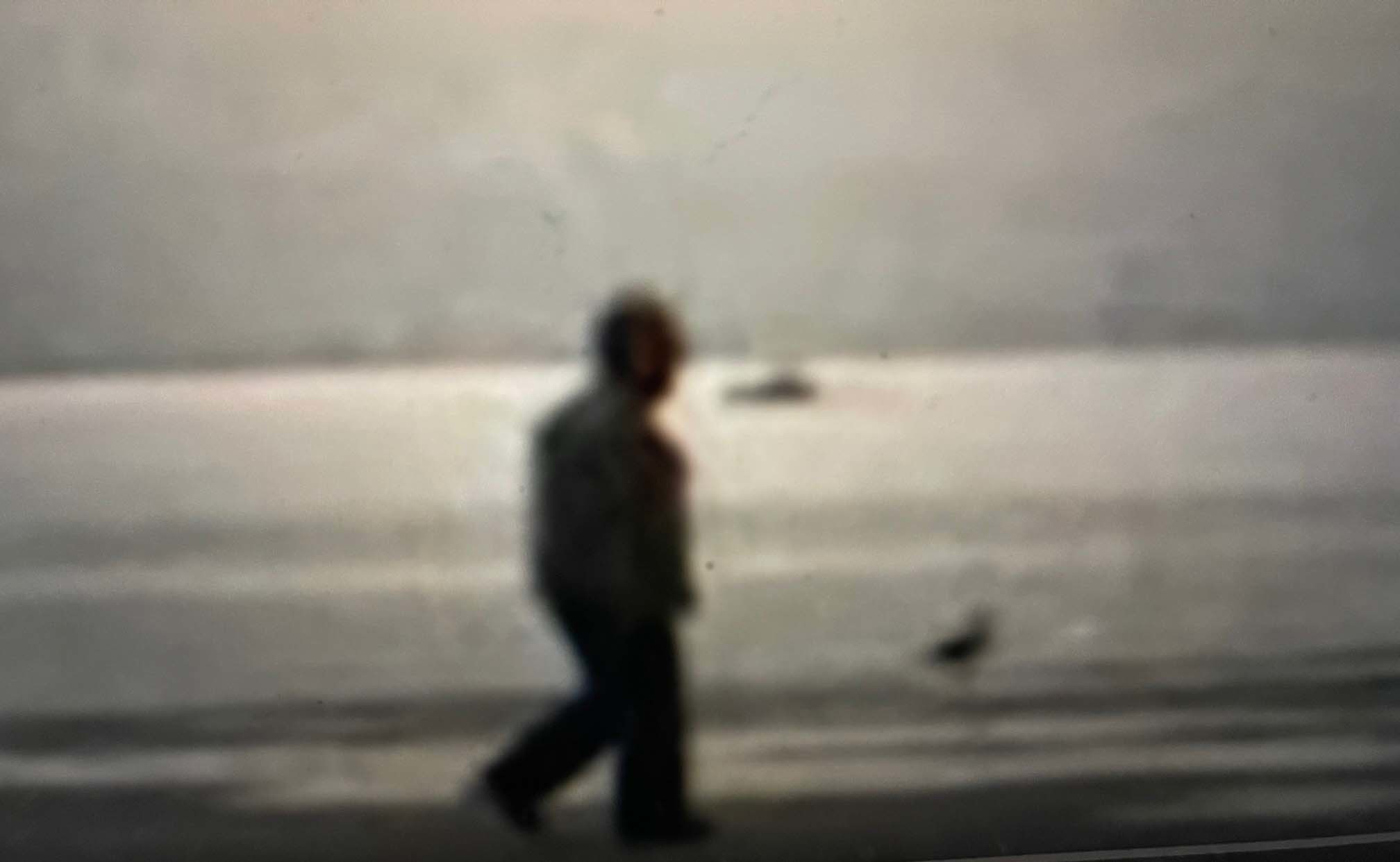A grayscale image captures a mysterious scene at the edge of the ocean. The sky, a medium tone gray, occupies the upper portion of the image, contrasting with a lighter stretch of water that spans horizontally from the center left to the center right. Off-center to the right, a large, indistinct object floats in the water, possibly a small boat. In the foreground, a fully shadowed silhouette of a person, clad in long pants and a jacket, walks from left to right along the sand. Just ahead of them, a bird dances near the surging ripple of a wave washing onto the shore. The lower edge of the image fades into a dark gray, enhancing the enigmatic and somber atmosphere.